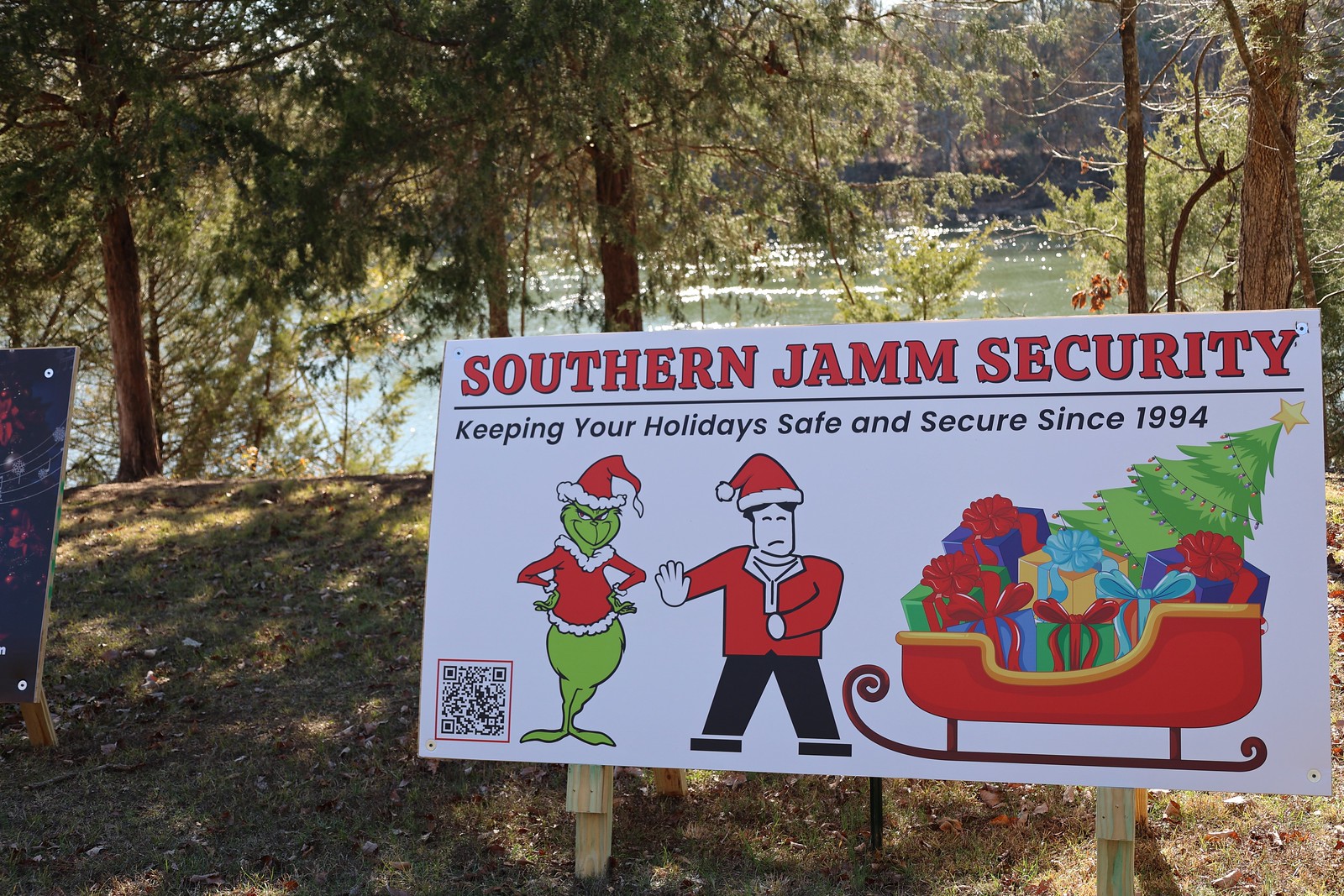The image features an outdoor advertisement resembling a ground-level billboard, supported by a couple of wooden frames and positioned in the middle to the right of the picture. The billboard itself has a white background and prominently displays "Southern Jam Security" in red text at the top, with "Keeping your holidays safe and secure since 1984" (not 1994) in black text below it, separated by a dividing line. In the bottom left corner, there is a QR code next to a colored, animated depiction of the Grinch from Dr. Seuss, dressed in a red Santa coat and hat. 

Adjacent to the Grinch is a black-and-white, animated image of a man also wearing a red Santa suit and hat, raising his arm in a gesture that suggests he is signaling the Grinch to stop. To the right of these characters is a large, red sleigh filled with presents and a green Christmas tree. The background reveals a serene river reflecting sunlight, framed by a dense border of green trees and extending to more trees on the distant shore. The billboard stands on a patch of brownish-green grass, completing the festive and secure holiday scene.